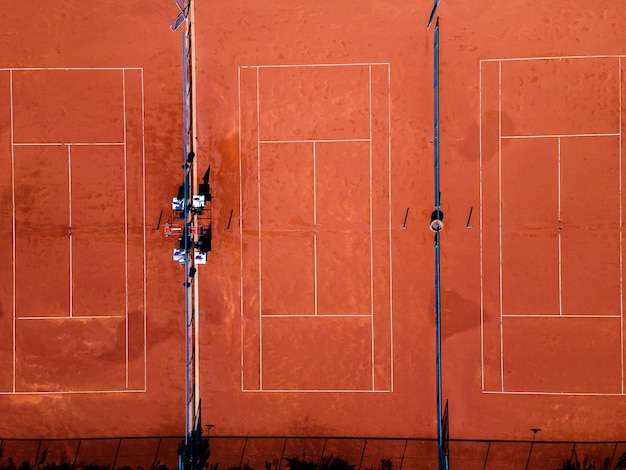This color photograph, captured in landscape orientation from a high vantage point such as a balcony or drone, presents an aerial view of three side-by-side red clay tennis courts. Each court is of identical size and shape, featuring the usual white play lines marking the court spaces. Notably, the central court is fully visible while the left and right courts are partially cut off. Separating the courts are blue fences or dividers, and a very tall perimeter fence surrounds the entire area, likely for spectator safety and ball containment. The leftmost court shows signs of wear and tear, with some play lines noticeably faded from use. Benches are positioned along the fences separating the courts, providing seating for players or spectators. The photograph captures the realistic, detailed essence of the courts from an elevated perspective, emphasizing the layout and condition of the facilities.